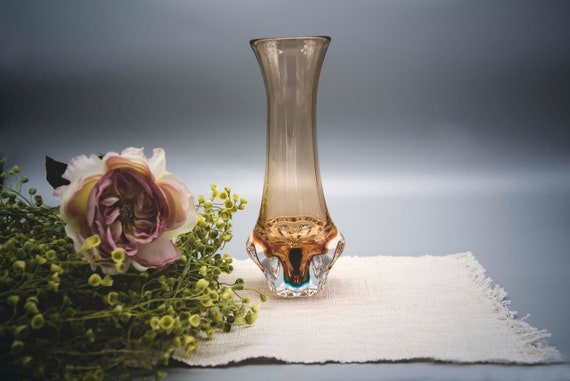The image is a detailed photograph taken indoors, exhibiting a tall, narrow vase with a unique design. The vase features a light orange-brown tint, permitting partial visibility through it. The upper section maintains this translucent hue, while the bottom transitions into a white shade adorned with a slight blue band and an orange interior, contributing to its jewel-like, reflective quality.

The vase is positioned on a white cloth, which is slightly frayed at the edges and spread out across the bottom right of the frame. To the left of the vase sits a vibrant bouquet. The bouquet prominently features a large rose-like flower with white outer petals and pink-tipped inner petals, which deepen to a cream color towards the center. Accompanying this main flower are long green stalks with small greenish-yellow buds adorning their tips. 

The background of the photograph is an interesting grayscale gradient that starts as a medium gray at the top, gets darker towards the middle, and then transitions into a highlighted white band before returning to medium gray at the bottom. This background further enhances the delicate shadows and the play of light and reflection within the scene, giving the entire composition a calm yet elegant appearance.